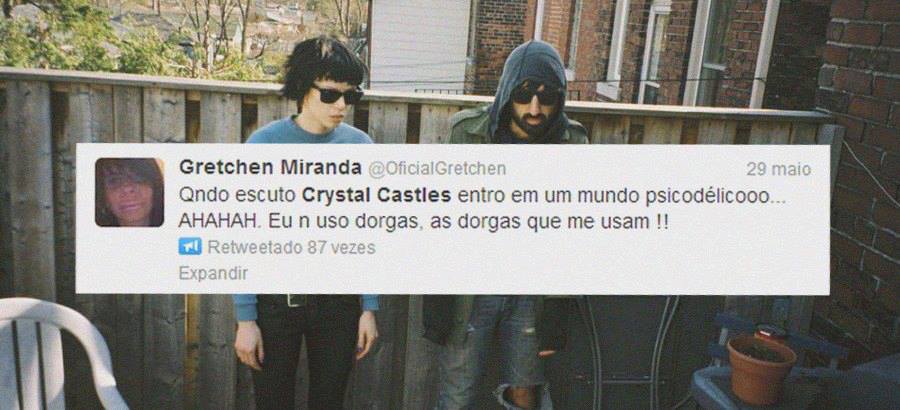The full-color photograph, taken outdoors during the daytime, features a setting that combines elements of nature and architecture. In the upper left corner, a few green trees and leaves are visible, adding a touch of greenery to the scene. On the right side, the brick wall of a building with double-hung windows framed in white provides a backdrop. The lower right corner showcases a small flower pot, while the lower left corner has a white plastic chair, indicating a casual, possibly residential setting.

In front of a brown wooden fence, two individuals stand side by side. Both are wearing sunglasses; one has a beard and wears a hoodie, while the other has curly hair, their gender not immediately clear. The photo appears to be taken on a balcony or an outdoor space associated with an apartment or townhouse.

Superimposed on the photograph is a social media post, evidently from Twitter, by Gretchen Miranda (@OficialGretchen). Her profile picture, positioned to the left within the overlay, shows a woman who appears to be around 35 years old. The tweet, dated the 29th of May, is written in Spanish and mentions "Crystal Castles," displaying some enthusiasm with phrases such as "entro em mundo psicodélico... ah ha ha ha e eu não uso drogas, as drogas que me usam," followed by two exclamation marks. The tweet has been retweeted 87 times, indicated by "Retweetado 87 vezes," and includes an option to "Expandir" or expand.

This multi-layered image captures a moment in a visually rich outdoor setting, detailed with personal elements from social media.